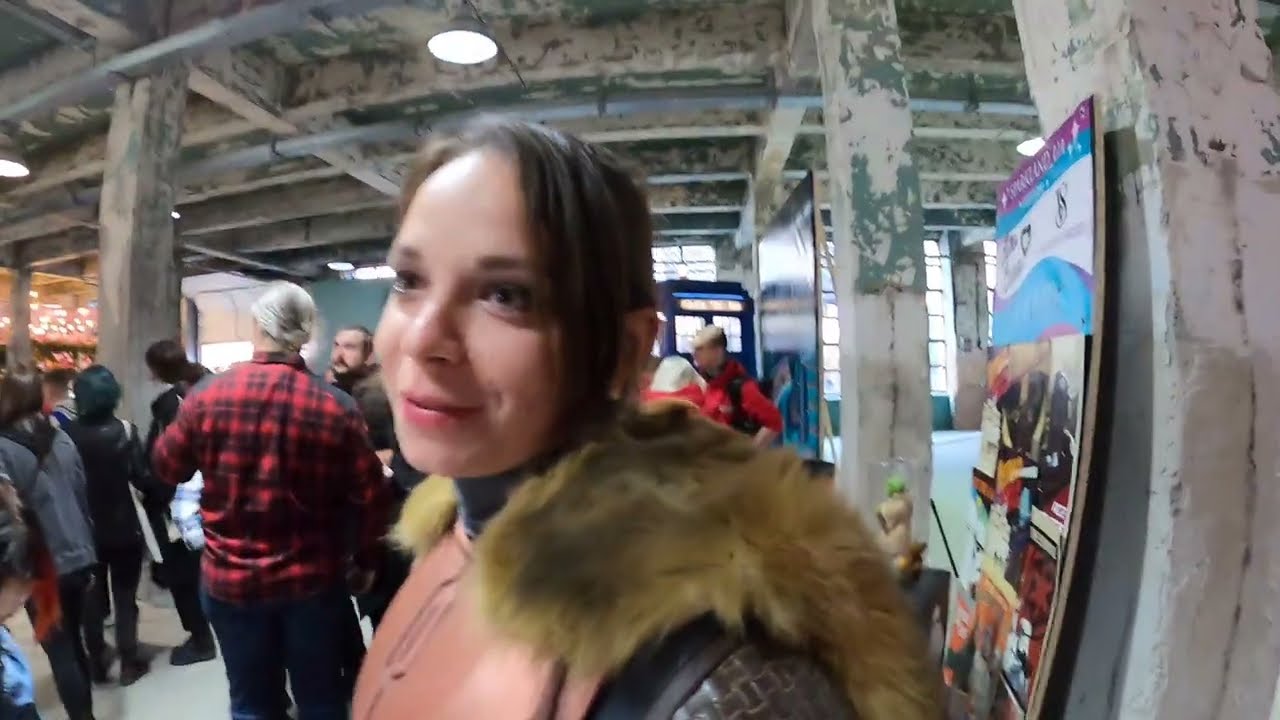Set inside a repurposed old warehouse with tall ceilings and white square columns showing signs of peeling paint, the photograph captures a casual event where people are gathered in clusters, possibly chatting or waiting for something to begin. The warehouse, which has round ceiling lights and sunlight streaming in through windows, features a booth that might be used for food, drinks, or purchasing items. Prominently in the foreground is a young woman with fair skin and short dark brown hair, wearing a jacket with a furry hood or collar. She stands out as she smiles, her lips adorned with lipstick, while looking slightly to her left. Behind her is a man with gray hair, facing away, dressed in a red and black plaid shirt. The ceiling, a mix of green and gray chipped paint with exposed beams and rafters, adds to the vintage atmosphere. Onlookers can see posters and panels with graphics and pictures adorning the background walls.